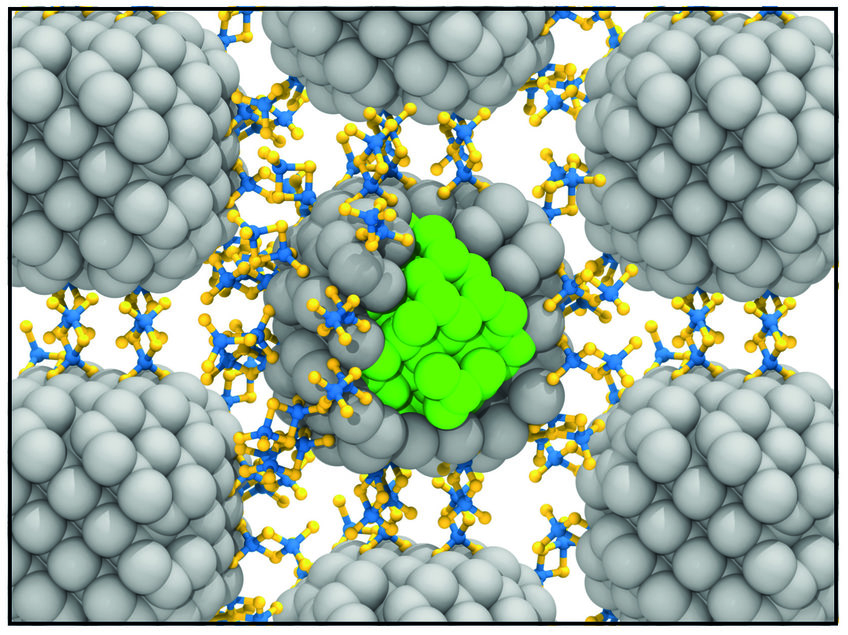The digitally synthesized image depicts a complex chemical compound or molecular structure, featuring a central sphere surrounded by six additional spheres, all composed of numerous smaller gray spheres. The central sphere has a core of similarly-sized but green-colored spheres, enhancing its distinctive appearance. Attached to the outer surface of each sphere are small blue matrices with yellow protrusions, which act as interconnections between the spheres. These connectors intricately link all the spheres together, resembling chemical bond representations. Each of the seven main spherical clusters appears to be identical in structure, with the central sphere standing out due to its green core. The arrangement forms a visually complex network against a plain white background, likely illustrative of an elaborate molecular or atomic compound often seen in educational materials such as textbooks or scientific presentations.